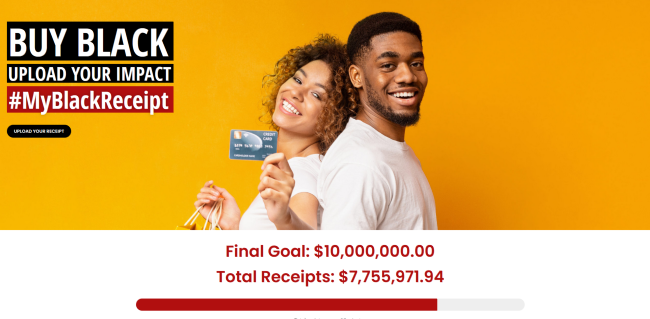In this vibrant, mustard-yellow horizontal rectangle, we see a detailed image featuring a man and a woman, both dressed in simple white t-shirts. The man, characterized by his very short, tightly curled black hair, slight mustache, and beard, sits back-to-back with the woman. The woman, who has long, voluminous curly hair, is seen holding a credit card in her left hand and is resting her head back against his. Her head is slightly tilted upwards, adding a sense of relaxed intimacy to the scene.

In the upper left corner of the rectangle, there are several smaller black and red rectangles with important messages. The largest black rectangle displays the words "BUY BLACK" in bold white capital letters. Directly beneath it, a smaller black rectangle bears the text "UPLOAD YOUR IMPACT" in the same white font. Following this, a red rectangle with white writing bears the hashtag "#MYBLACKRECEIPT."

Further down, there is an indication of a financial goal and current progress: "Final Goal: £10,000,000," with the current total reading precisely "£7,755,971.94." This caption highlights the significant campaign aimed at encouraging economic empowerment within the Black community.